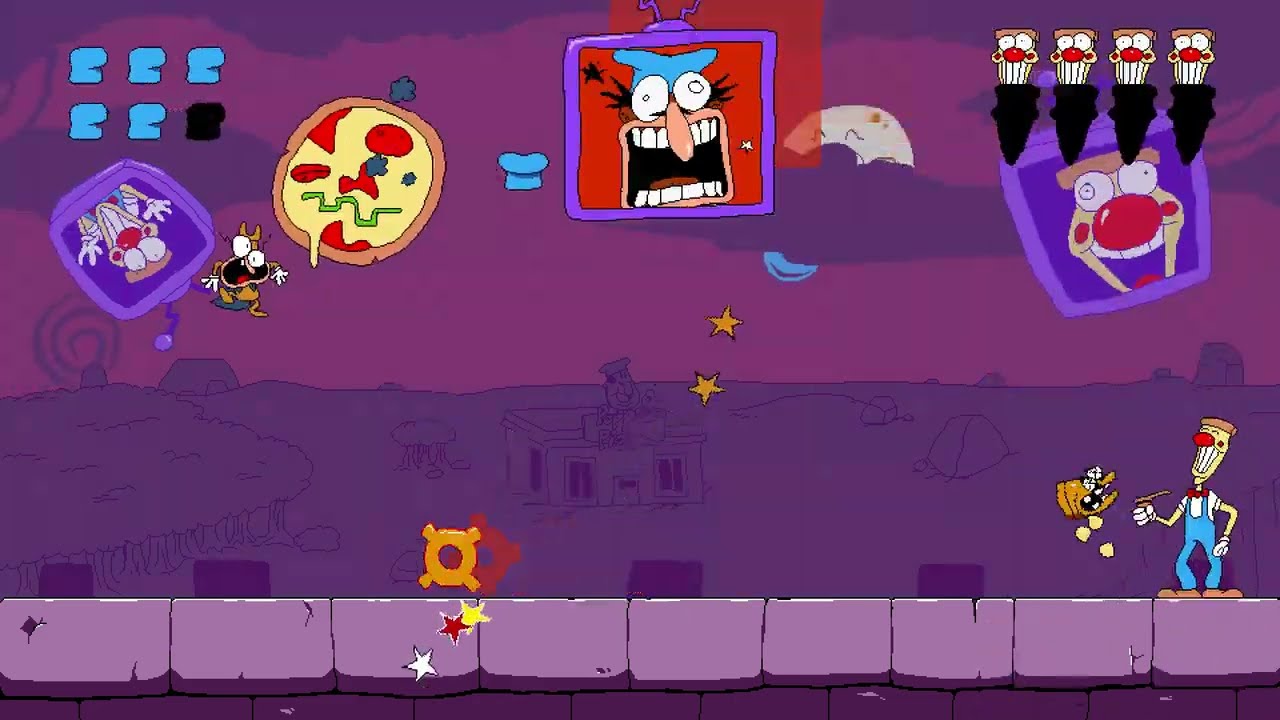The image is a screenshot from a colorful and highly animated video game scene with a distinct purple hue throughout the background. The sky features a gradient of medium to dark purple, with the ground depicted in a darker purple shade. In the background, a faint outline of a house is visible. At the bottom of the image, there's a horizontal walkway made of light brown bricks.

In the bottom right corner, the main character stands out with a large, exaggerated smile. He has yellow skin, a wide mouth, and a red nose, and is dressed in blue overalls over a white shirt. He appears to be looking up at an odd item hanging in the sky, which resembles a bag of potato chips with eyes atop it and potatoes falling down.

In the top middle section of the image, a large face is visible, characterized by a long nose, wide open mouth showing all his teeth, large white eyes, and a blue hat. This face is set against a bright red background. Surrounding it are fragments of other animated faces and objects, including pizza slices and dog-like faces. The upper left corner displays two horizontal rows of what look like blue hamburger halves and another floating pizza slice.

Additionally, there are scattered animated faces with big white eyes and red noses throughout the top portion of the image, and orange and multicolored stars appear among the purple blocks at the bottom. The entire scene is vibrant and dynamic, packed with various quirky characters and elements floating or seemingly in mid-fall, giving an overall lively and interactive video game feel.